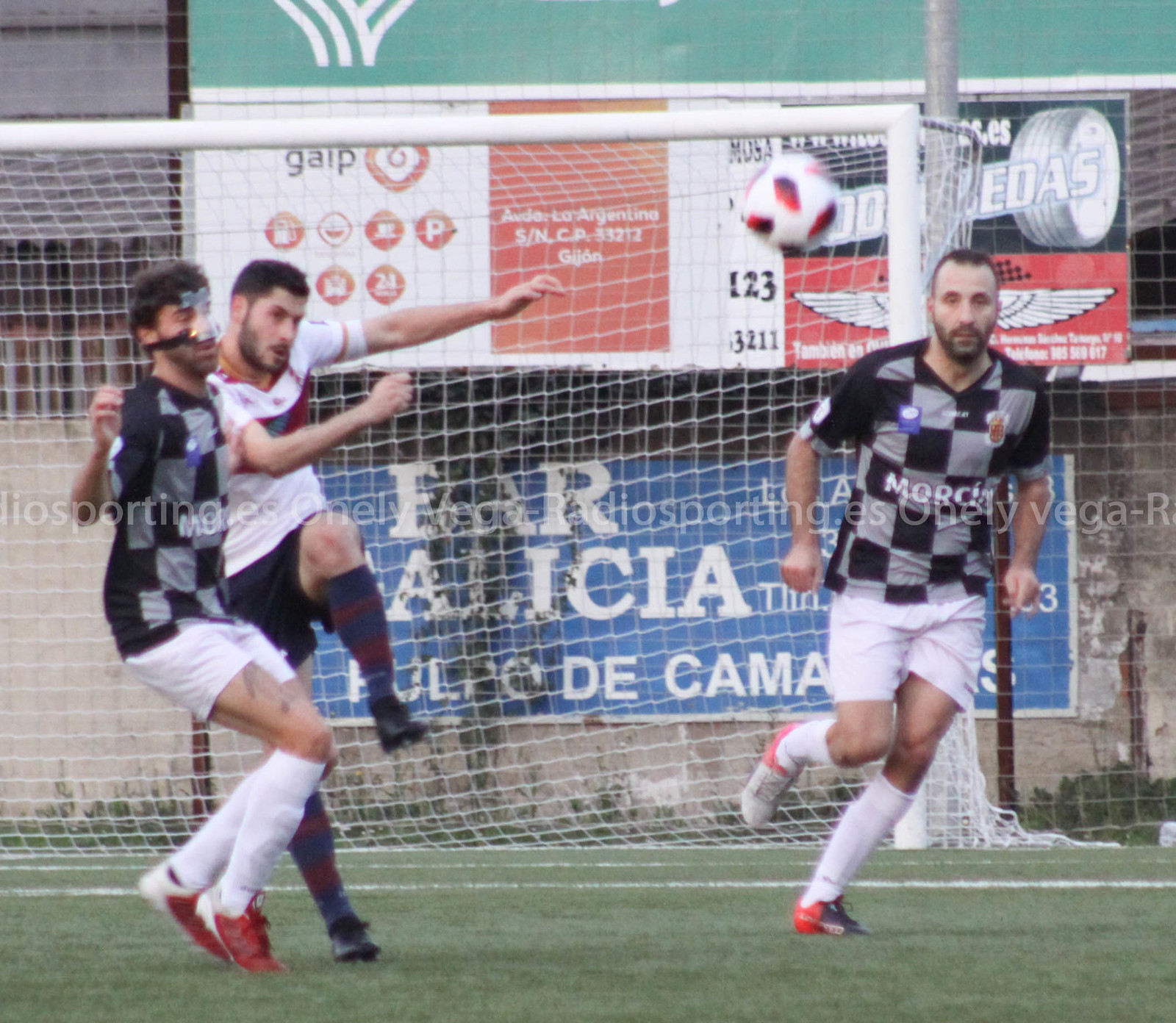In the image, taken during an intense soccer match, three men are captured mid-action on a green soccer field in front of a white goal post with netting. The ball, white with black and red patterns, is suspended in the air above their heads. Two players are dressed in black and silver checkered jerseys, white shorts, and white socks, both running toward the ball with red and white cleats. One of them, on the left, is distinguished by a face guard, possibly for protection or due to a prior injury. The other player wears a short beard. The third man, dressed in a white uniform paired with blue shorts, blue and red socks pulled up to his knees, and black soccer shoes, is leaping impressively high in the air, attempting to reach the ball. Behind them, various banners line the background, including a standout advertisement featuring a car tire with eagle wings below it. The scene unfolds near the goal, capturing a dynamic moment of the game.